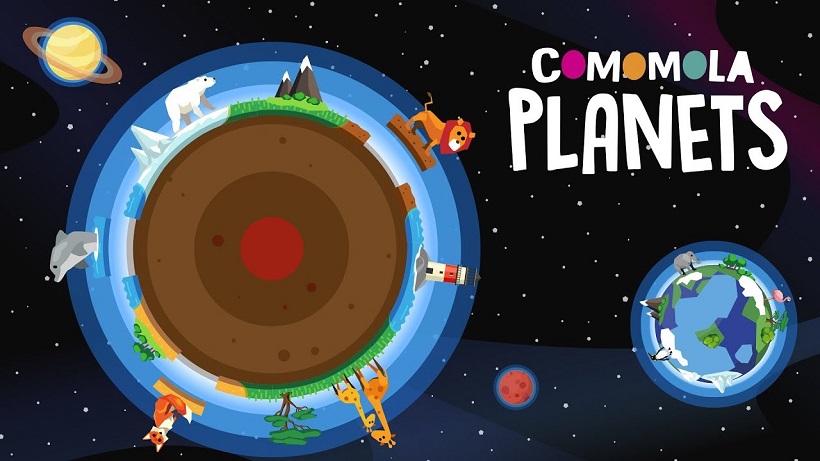The image depicts a digitally-created cartoon illustration featuring a colorful cosmic setting. Against a black background dotted with white stars, the foreground showcases four distinct celestial bodies. In the top left corner, there is a yellow planet encircled by a brown ring, reminiscent of Saturn. Centrally located, the largest planet is a blue sphere outlined in various shades of blue, brown, and a bright red core, teeming with diverse animals including lions, giraffes, foxes, whales, polar bears, trees, and even a lighthouse. To the bottom right, another Earth-like planet appears, characterized by vibrant blues and greens. Further to the left of this smaller planet is a small red celestial body. The top right corner contains the text "Common Yule Planets," with the letters "C-O-M-O-M-O-L-A" displayed in pink, orange, and green. The abundant colors present include red, brown, green, tan, gray, white, orange, yellow, dark red, dark blue, fuchsia, dark teal, and maroonish red, accentuating the vibrant and whimsical theme of this cosmic illustration.